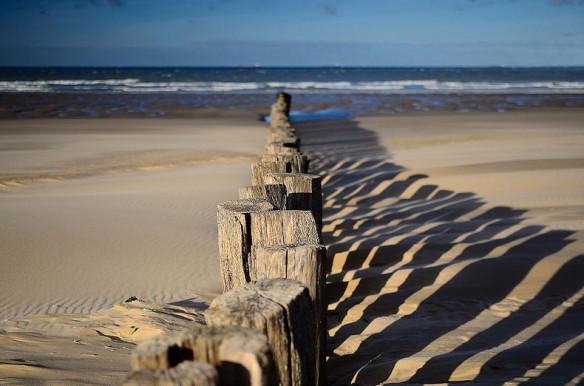The image showcases a serene, uninhabited beach under a vibrant blue sky. Centered in the picture, a row of weathered wooden posts, some visibly cracked and split, lead towards the ocean, casting distinct shadows to the right, indicating sunlight from the left. The shadows of these posts are beautifully cast onto the sand, adding to the tranquil atmosphere. The sand, a beige color with ripples and a slightly dirty appearance, flanks either side of the posts. In the distance, the ocean's blue waters are capped with white waves crashing gently onto the shore. Despite some blur in the background, the overall scene captures a simple yet stunning coastal landscape.